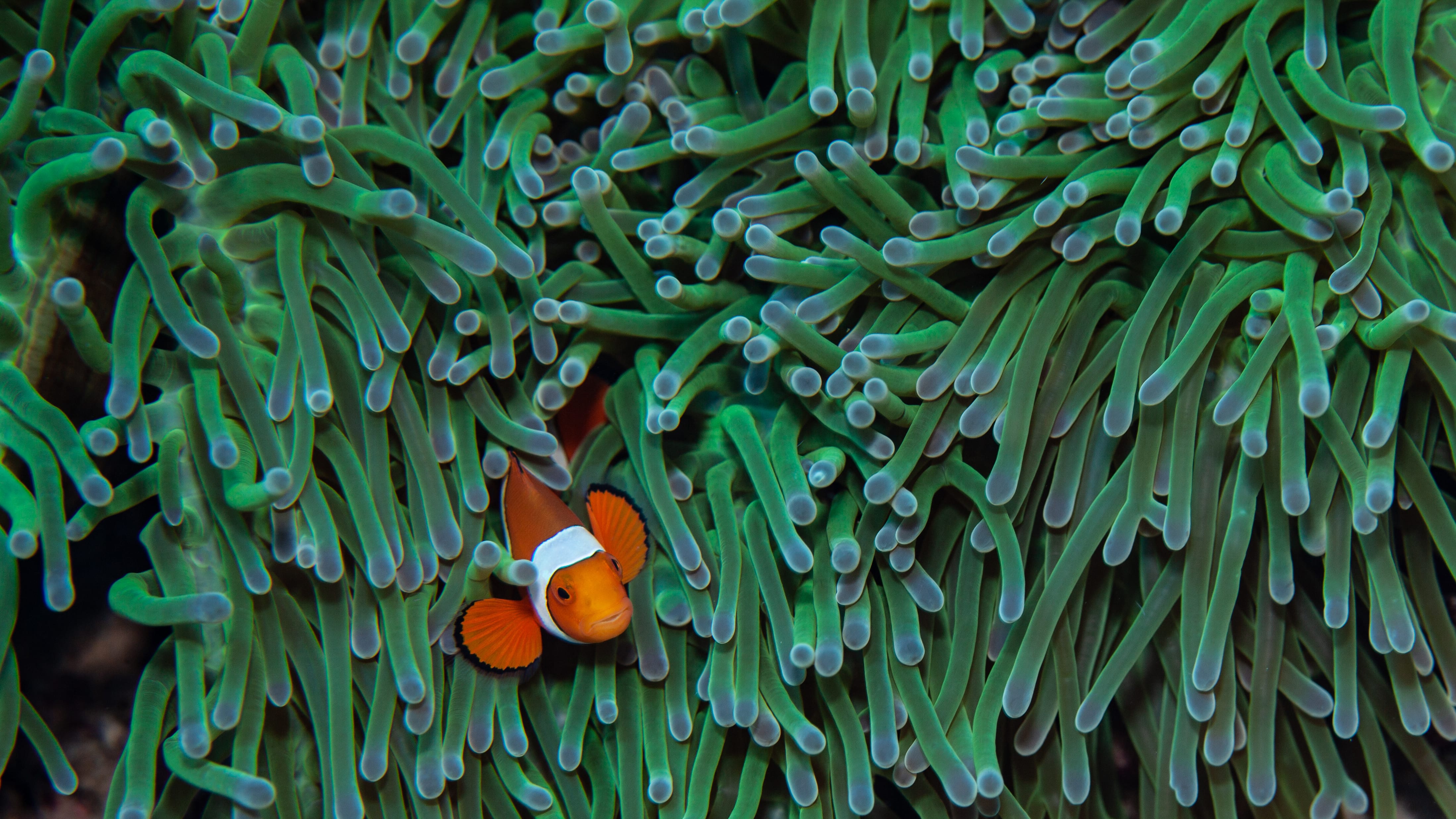The image depicts a vibrant underwater scene featuring a clownfish, easily recognizable by its striking orange body and a distinctive white stripe encircling its neck. The clownfish is positioned in the bottom-left quadrant of the picture, swimming with its tail slightly elevated. Its fins, bordered in black, are extended outward as if in motion. It is nestled amongst a dense array of green, worm-like ocean plants that dominate the scene. These plants are slender and finger-like, with tips resembling gray Q-tips, though they also display yellow or brown tinges at the ends. The majority of these plants, directed downwards, create a textured and lively backdrop that encapsulates the vivid marine habitat. The overall scene is reminiscent of popular depictions from films like "Finding Nemo," capturing the intricate and colorful dynamics of underwater life.